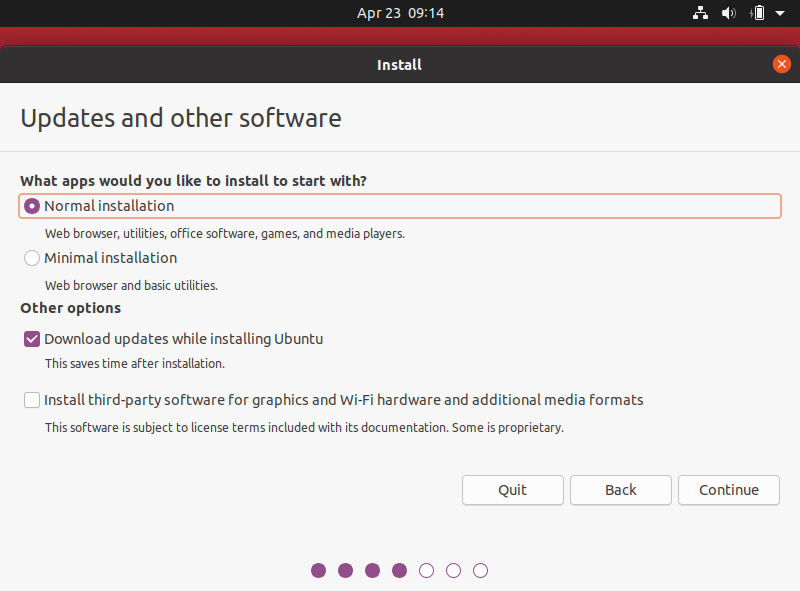**Detailed Caption:**

This screenshot captures the 'Software & Updates' page on a user's device, potentially a laptop or tablet. At the top, the device displays essential system information, including the date "April 23rd" at "9:14" centered on the screen. On the right side, indicators show a full battery icon and a volume setting, accompanied by a downward arrow for additional options.

The main section of the screenshot focuses on the 'Install' tab, emphasized by a red and gray bar and an orange circle with an 'X' on the right side. Under the header 'Updates and Other Software,' the instructions for selecting installation preferences are presented. 

The first section, titled 'What apps would you like to install?', highlights two bullet points:
1. **Normal Installation** - This option has an orange box around it and is filled in, indicating it is the current selection.
2. **Minimal Installation** - The alternative choice available to the user.

Below this, a bolded section labeled 'Other options' lists two additional settings with checkboxes:
- The first checkbox, marked as selected, reads, “Download updates while installing Ubuntu.”
- The second checkbox reads, “Install third-party software for graphics and Wi-Fi hardware, and additional media formats,” which is currently not selected.

At the bottom right of the screen, navigation buttons include 'Quit,' 'Go Back,' and 'Continue,' providing the user with the choice to exit the installation process, return to the previous step, or proceed further.